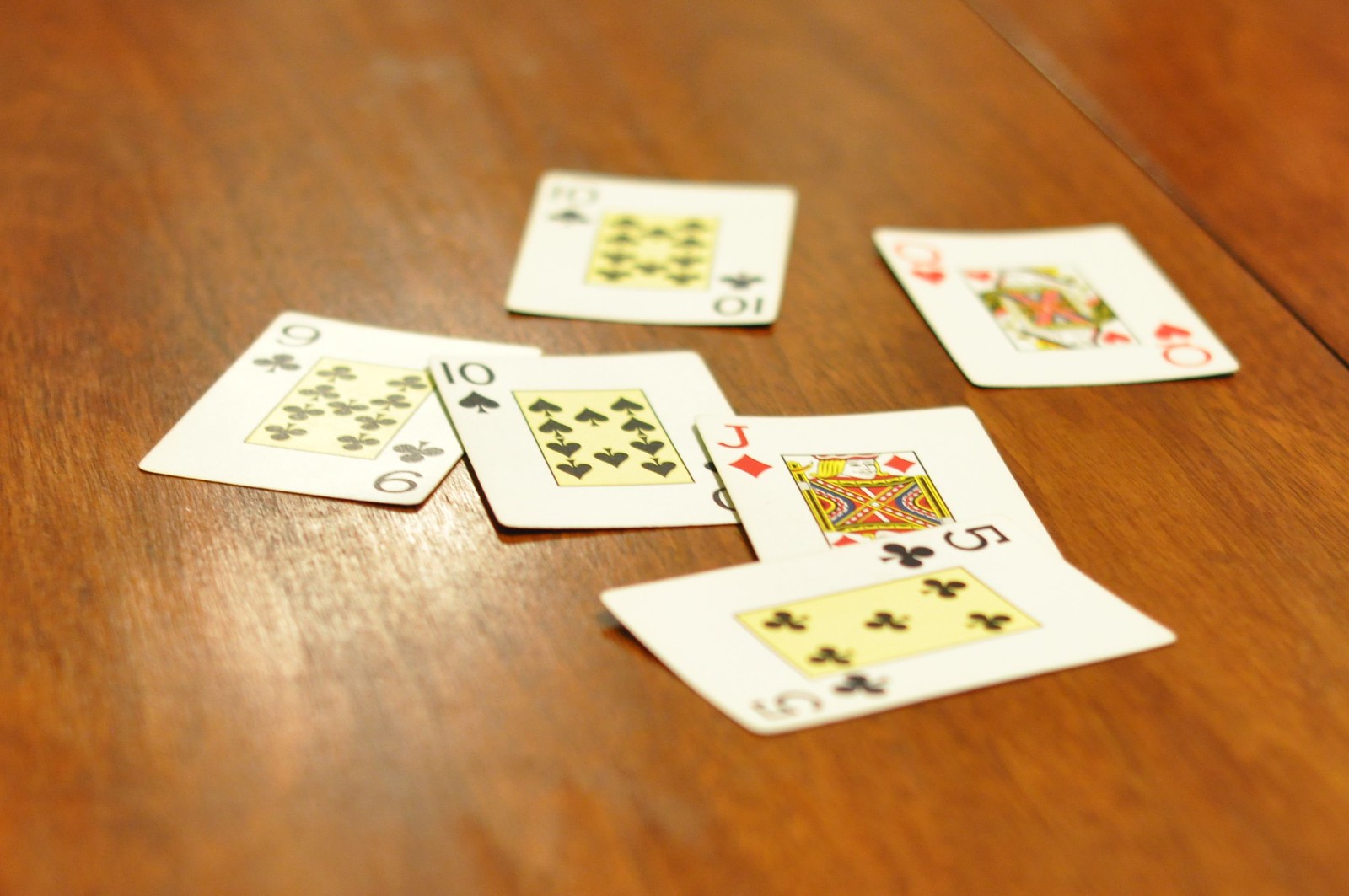A detailed description of the image:
This photograph captures six playing cards laid face-up on a medium-colored wooden table with a reddish hue. The cards displayed are the ten of spades, nine of clubs, ten of clubs, jack of diamonds, five of clubs, and queen of hearts. The queen of hearts and the ten of clubs are slightly set apart from the others, while the nine of clubs, ten of spades, jack of diamonds, and five of clubs are touching each other.

Each card is presented on a white background, and centrally, there's a square rectangular section with a pale yellow background. Within this section, the clubs and spades symbols are displayed in black. Both the jack of diamonds and the queen of hearts feature illustrations of their respective characters within a central rectangular area on a white background. Additionally, each card has its number and corresponding symbol displayed in the top left, top right, and bottom right corners.